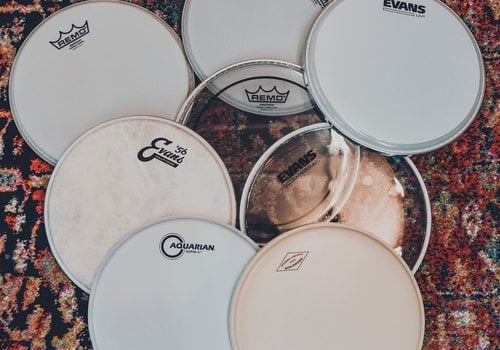The photograph captures seven round drum heads arranged on a multi-colored, oriental-style tapestry. The tapestry features a blend of black and red, suggestive of a 70s pastel style, with the left side predominantly black and the right side mainly red. Each drum head is marked with a brand: several are labeled Remo, some say Evans 56, and one is marked Aquarian, positioned at the bottom left. The drum heads form a semicircular pattern, with slightly overlapping edges, allowing each one to be distinctly visible. Among the drum heads, two stand out as transparent, both centrally located, while the rest are opaque white. Notably, most of the drum heads appear unused and in good condition, except for one in the center which shows slight signs of use with a grayer appearance.